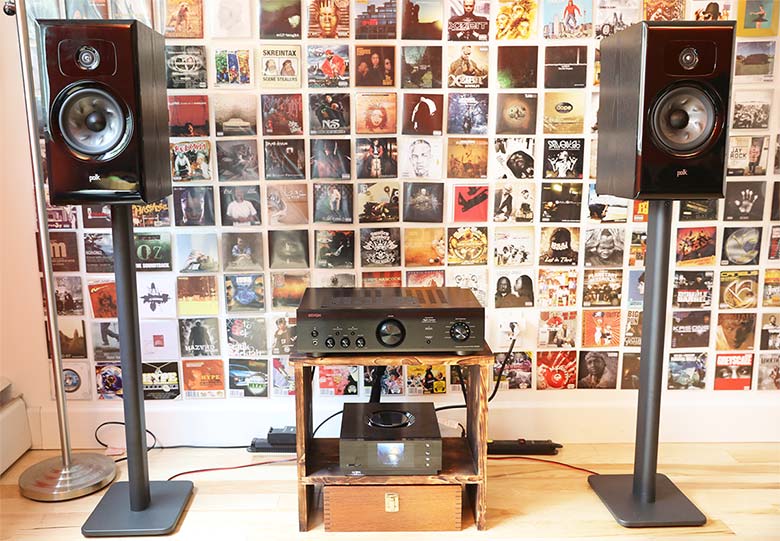The image depicts an elaborate music listening setup in a room with a hardwood floor. At the center, there is a brown wooden stand featuring a shelf and a drawer. On the stand sits a stereo receiver, identifiable by its silver color and volume and bass dials. Flanked on either side of the stand are two black Polk Audio speakers mounted on gray pole-like stands. The speakers have a detailed design that includes silver and gray accents, with some text at the bottom. The wall behind this setup is white and adorned with a vivid collage of album covers, predominantly from hip-hop artists such as Nas, The Notorious B.I.G., and Lauryn Hill. The artwork covers the entire wall, providing a colorful and thematic backdrop. Additionally, there is a lamp on the left side of the room, and several wires and plugs are visible around the middle setup, enhancing the authentic and functional vibe of this cozy music corner.